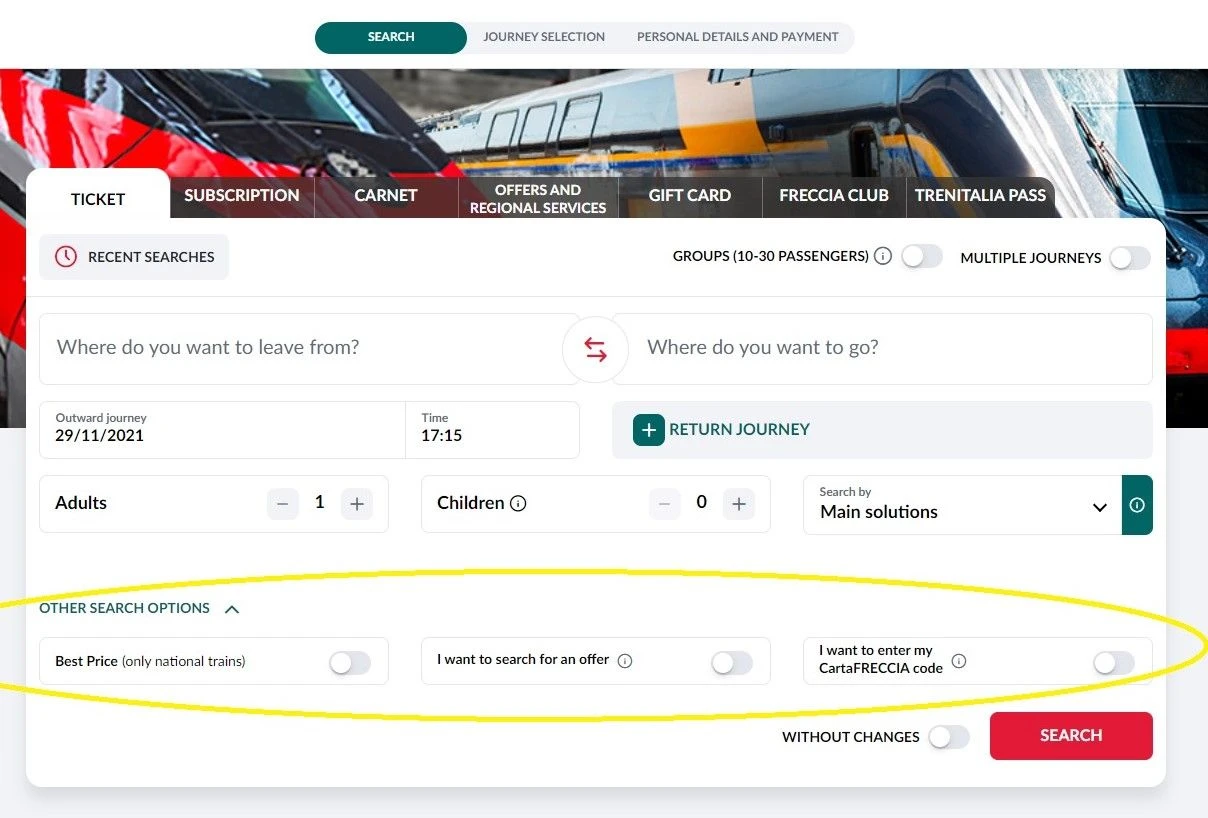A screenshot of a travel booking website, displayed in a metro-themed interface, serves as the focal point. At the top of the page, three primary navigation buttons are visible: "Search and Journey Selection," "Personal Details," and "Payment," with the "Search" section currently selected. Below this navigation bar is a visually appealing image featuring two sleek and modern subways; one is predominantly blue while the other is red.

In the foreground, the information input section for planning a journey is prominently displayed. Fields to be filled include "Outward Journey," specifying departure time, departure location, and destination. Additional options allow for entering the number of adults and children traveling. 

The page also features several selectable sections such as "Subscription," "Carnet," "Offers and Regional Services," "Gift Card," "FrecciaClub," and "Freccia." Circles have been drawn around different search options, emphasizing their availability. The option to sort search results by the best price is highlighted, suggesting a user-centered approach to finding the most economical travel options.